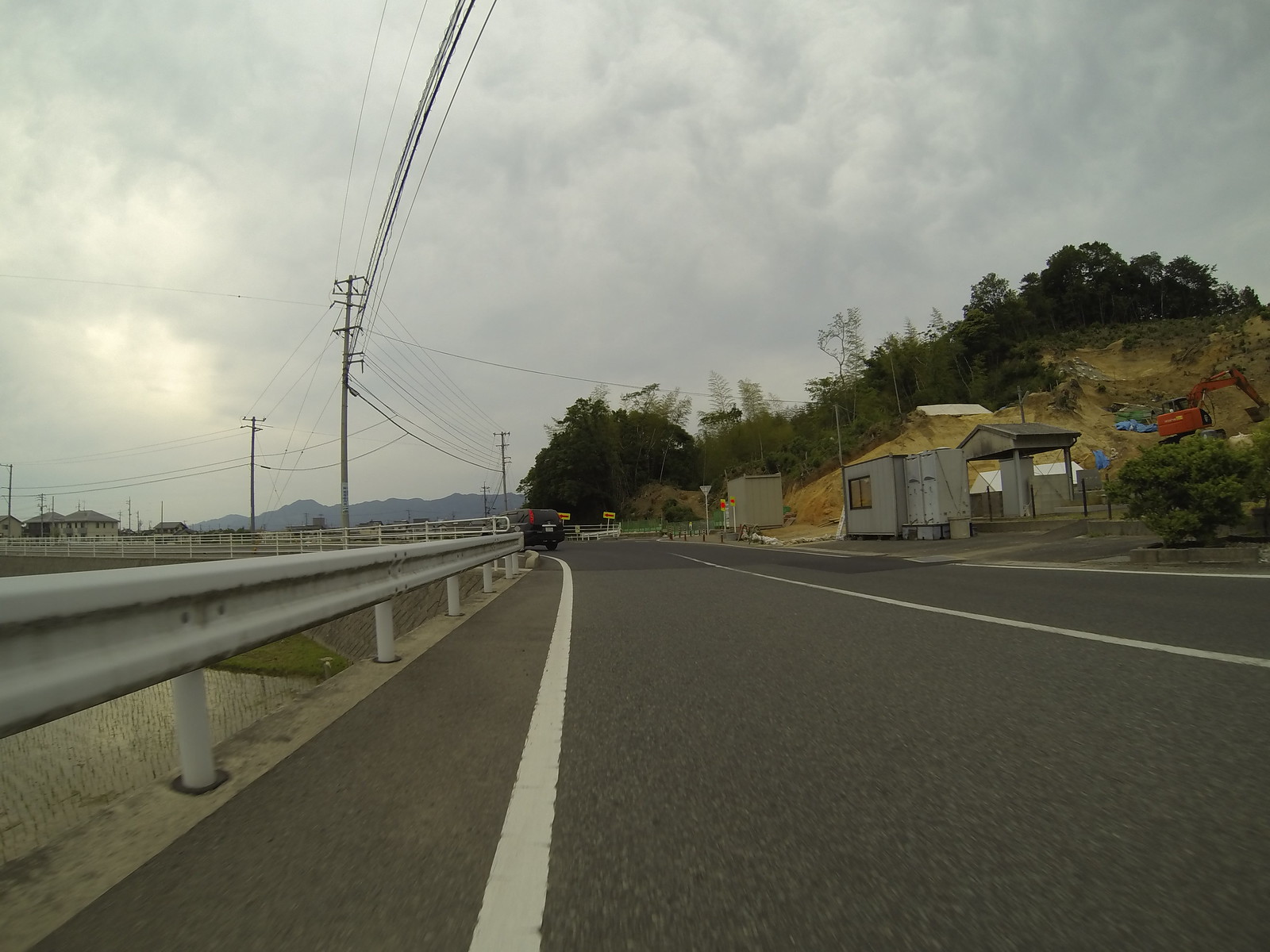This image depicts a stretch of a highway or major road. On the left side, there are metal guardrails designed to prevent vehicles from veering off the road, possibly into a lower level or over a bridge. In the foreground, a car appears to be making a left turn onto another road, or perhaps the highway itself curves leftward at this point. The road consists of two lanes, and the photo is taken from the left lane by someone inside another vehicle. The image is sharp and free of motion blur, suggesting that the vehicle from which the photo was taken is either stationary or moving very slowly.